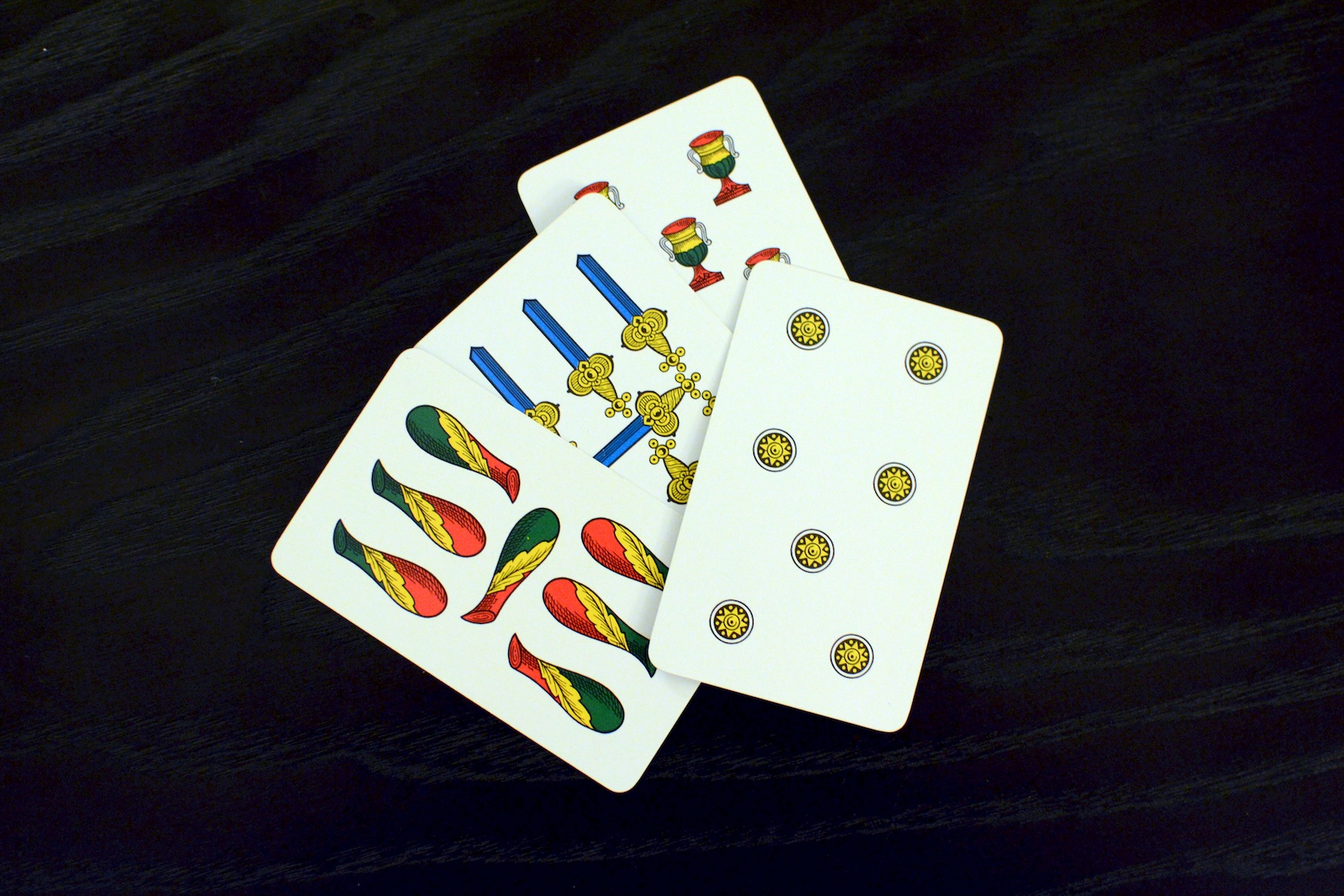A photograph captures a black wooden table adorned with a visible lighter black wood grain. On the table, there is a close-up arrangement of four tarot cards. The foremost card, slightly rotated to the right from a vertical orientation, features seven small gold sun symbols set in circles against a white background. Positioned to the left and partially behind it, another card displays seven intricate vases. These vases are adorned with a gold leaf pattern running diagonally through their centers, with alternating sections of green and red. Some vases have green at the top and red at the bottom, while others are the reverse.

Further back and oriented similarly, three-quarters of another card is visible, showcasing five symbols. These symbols resemble swords with blue blades and gold handles. The rear card, mostly obscured, depicts goblets. Four goblets are discernible, each with a red interior, dual silver handles, and adorned with two gold bands, a green lower section, and a red base. The meticulous details of the symbols and the textured table create a rich, layered visual.